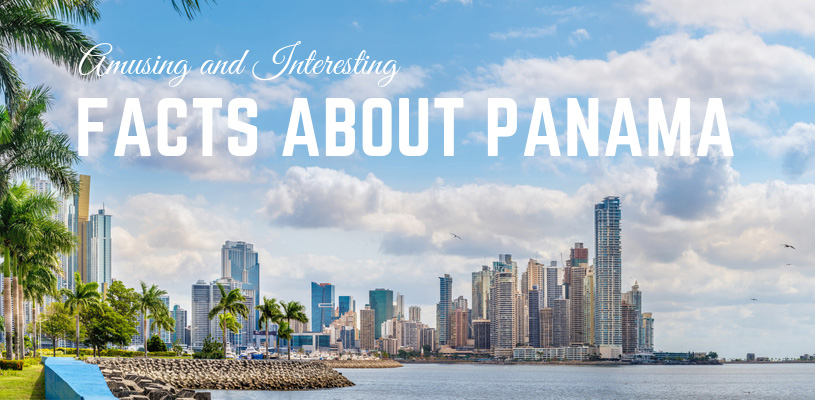A stunning daytime aerial photograph showcasing the vibrant cityscape of Panama City, Panama. The layout of the city resembles a peninsula, with the ocean curving gracefully around it. In the foreground, there is a sandy beach with visible patches of rock and sand, dotted with around eight to ten palm trees. A small blue object, possibly a docked boat, can be seen near the beach. The city skyline is dominated by approximately 40 to 50 tall buildings, including several towering skyscrapers. One prominent skyscraper, second from the right, stands out due to its considerable height. The sky above is mostly clear, with a few puffy clouds, and the tranquil waters surround the city, reflecting the calm and sunny weather. This captivating image, captioned with the phrases "Amusing and interesting" in cursive and below it, "Facts about Panama," offers a glimpse into the surprisingly extensive and bustling metropolis of Panama City.